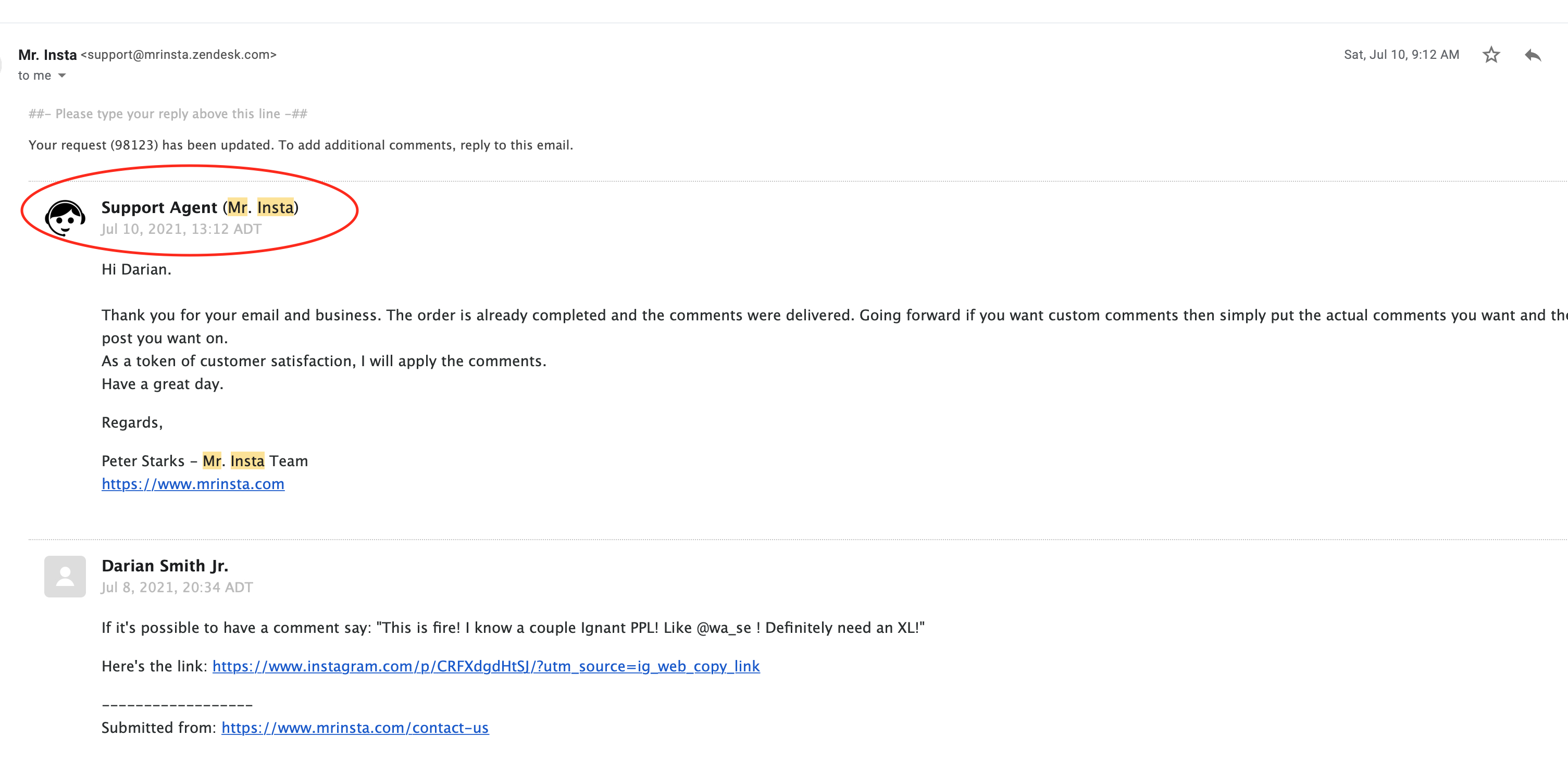Screenshot of an email exchange between Darian Smith Jr. and Mr. Insta Support Team.

The exchange begins with an email from Darian Smith Jr. sent on July 8, 2021. In this email, Darian inquires if it's possible to have a comment saying "This is fire 🔥. I know a couple ignant people like @wa_say definitely need an XL."

The email also includes a submission link for the convenience of the support team. Darian's message shows a clear request for a specific type of comment to be added to a post, reflecting his engagement with the customer support for tailored service.

The response from Peter Starks of the Mr. Insta Support Team, using the email address support@mrinsta.zendesk.com, is also shown. Peter's reply addresses Darian's inquiry and confirms that the order has been completed and the comments have already been delivered. He further provides guidance on how to request custom comments in the future, advising Darian to specify the actual comments and the desired post. As a gesture of customer satisfaction, Peter assures Darian that these comments will be applied.

Peter ends his email with a thank you note for Darian's business and a cordial sign-off: "Have a great day. Regards, Peter Starks, Mr. Insta Team."

The detailed correspondence highlights the personalized customer service approach of Mr. Insta and the proactive communication from their support team.